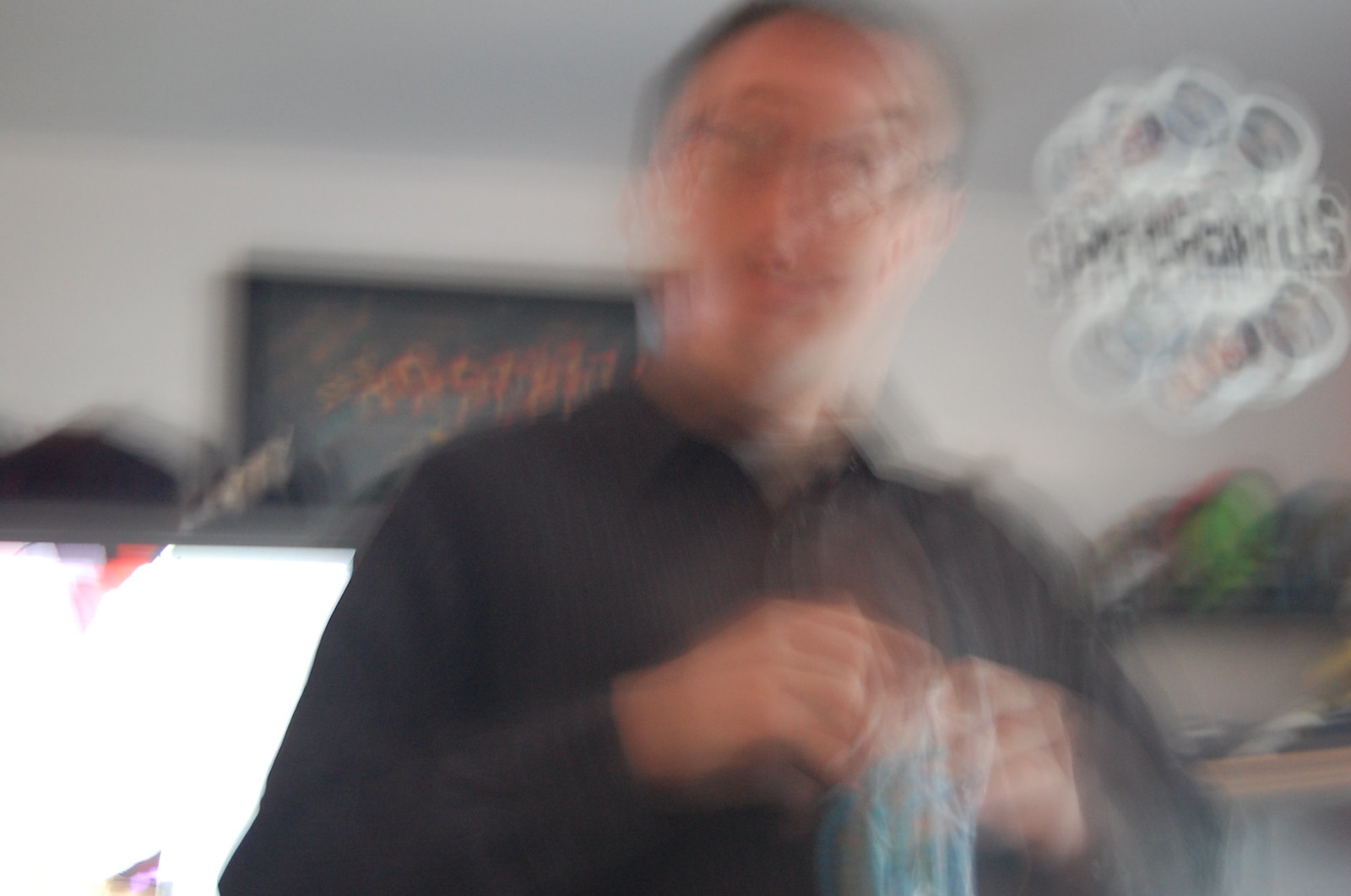Blurry and slightly distorted photograph of a man. He is wearing glasses and a black long-sleeve shirt. His hands are visible, holding a blue and tan object. The background reveals a white wall and ceiling. To the side of his head, there is a circular object with black text, and over his shoulder, another object with a black frame, black background, and orange font. A mirror with a dark brown or black edge and some light reflection is also visible behind him. Underneath the circular object, shelving with various items in shades of green, black, and white can be seen.